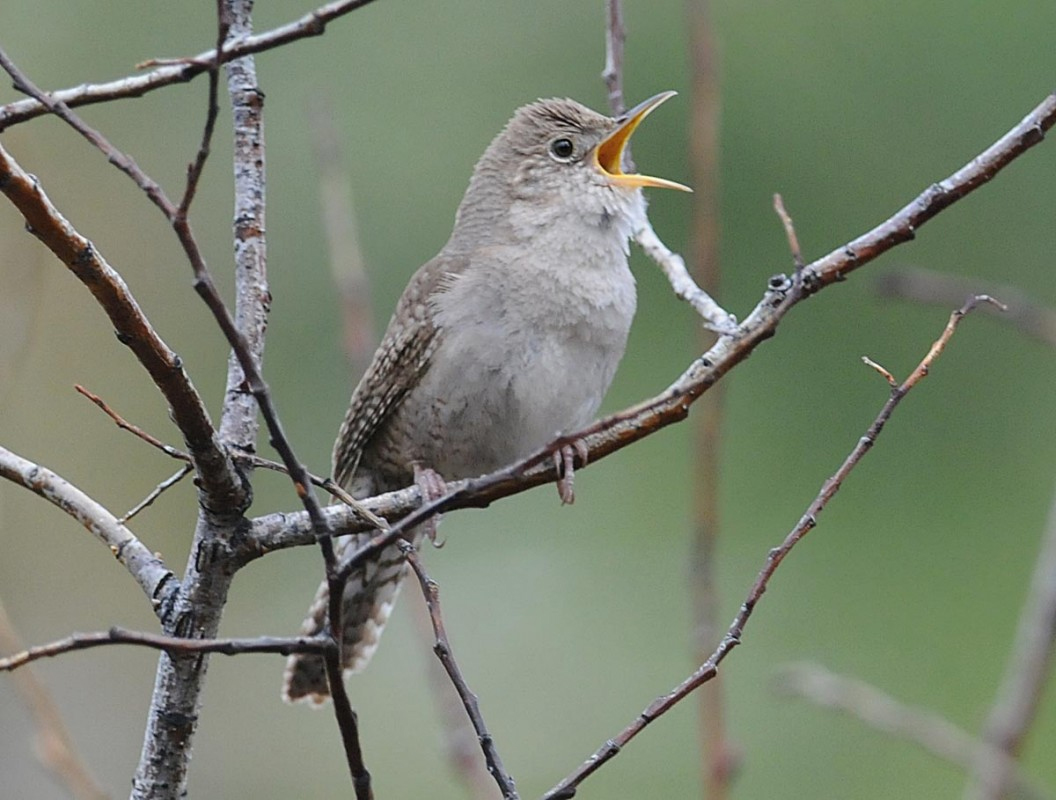In this detailed photograph, a small to medium-sized bird is perched perfectly on a thin, twig-like branch of a leafless tree. The bird, which is predominantly gray with light gray and medium gray speckled feathers, features a striking orange hue inside its long, pointed beak. Its dark, round eye is clearly visible, emphasizing its alertness. The bird's beak is wide open, suggesting it is either mid-chirp or waiting to receive food. The tree branches, devoid of leaves or buds, indicate a scene set in very late winter or early spring. Background details are blurred with hues of light green and white, enhancing the focus on the bird and its delicate perch. The bird's small, fleshy-colored feet grip the branch firmly, adding to the overall harmony of the image.